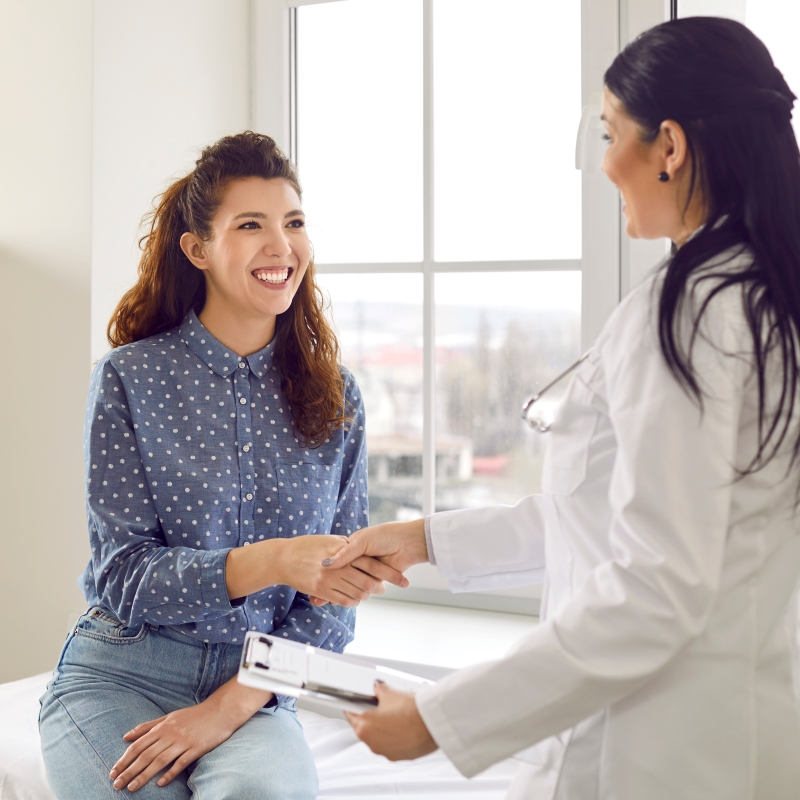This photograph captures a warm, professional interaction in a medical office featuring a doctor and her patient. The doctor, a young woman with pinned back, long flowing black hair, and a black circular earring, is positioned on the right side of the image. She has fair skin and is dressed in a long-sleeved white lab coat with a stethoscope around her neck, partially visible due to its silver sheen. In her left hand, she holds a clipboard with white papers and a black pen attached to it. Her right hand warmly shakes the patient's hand.

The patient, who is seated on an exam table with her legs crossed, faces the camera. She has light curly brown hair with copper highlights, also clipped at the back. She wears a slate blue long-sleeve button-up blouse adorned with white polka dots, paired with light blue jeans. She carries a cheerful expression as she looks at the doctor, her fair skin glowing with minimal makeup.

Both women exude a friendly and positive demeanor. The backdrop features white walls and a large, four-paned window with white window panes, through which a blurred landscape is visible, emphasizing the clean and professional atmosphere of the medical office.